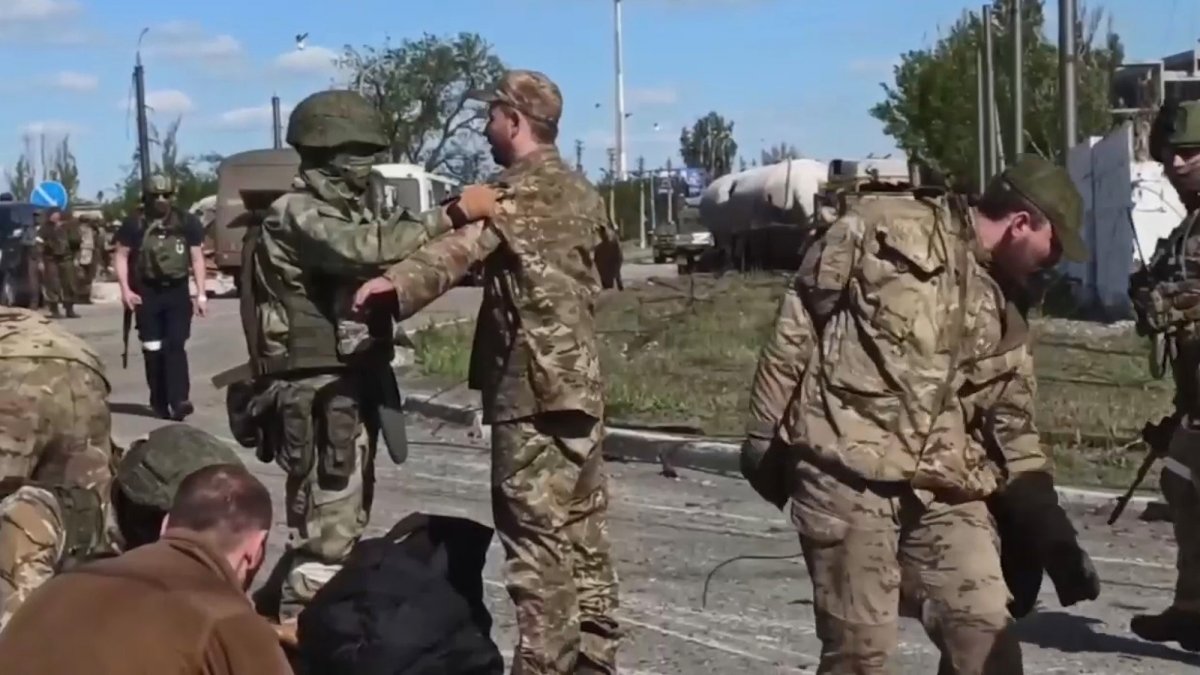In the image, a military checkpoint is set up on a cement roadway under a blue sky with scattered trees in the background. Central to the scene, a soldier clad in camouflage fatigues and a camouflage hat stands with his arms outstretched, being patted down by another heavily-equipped soldier wearing a helmet, face mask, and vest. To the lower left, a group of people, some in camouflage and one in a brown jacket, sit on the ground. On the right, another soldier in camouflage and a green hat bends over, while additional helmeted and masked soldiers are seen in the background. The narrow road, resembling a street flanked by buildings and possibly military vehicles, including a truck, creates a bustling backdrop of military activity. There's also a noticeable red sign and some loitering soldiers further emphasizing the checkpoint's scenario.